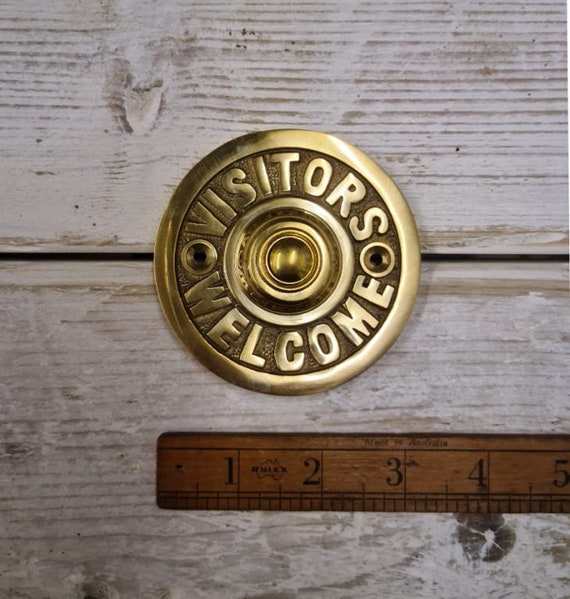The photograph is a vertical, full-color image staged indoors using artificial light. It showcases a round, brass-colored button with the words "Visitors Welcome" engraved on it. This button, resembling a snap typically found on clothing, is mounted on a whitewashed wooden surface. The button, which has a slight glow in its center, is affixed using two screws positioned to the left and right (east and west). Below the button lies a well-worn, dark brown ruler with black numbering, displaying measurements from 1 to 5 inches. The ruler, resting on a light wood table with visible grain, indicates that the button has a diameter of approximately 3 inches. The vertical black line running through the middle of the image is the seam between two wooden boards. This detailed setup presents a peculiar yet charming welcome ornament, blending elements of practicality and vintage aesthetics.